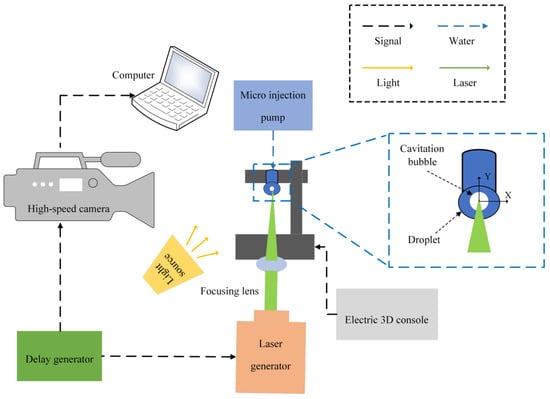The image is a detailed infographic illustrating the operation of a high-speed imaging and microinjection system. Starting from the top left, a labeled white laptop represents a "Computer," from which black dotted lines link downwards to a gray diagram labeled "High-Speed Camera." Adjacent to this camera, a green rectangle labeled "Delay Generator" connects via dotted lines, both to the left towards the high-speed camera and to the right towards an orange rectangle labeled "Laser Generator." From the laser generator, a green spike adorned with a gray ring, labeled "Focusing Lens," points towards a black frame structure hosting a blue lens, described as a "Micro Injection Pump." Central to the diagram, a section titled "Light Source" is included. To the right of this primary setup, several color-coded arrows illustrate different components and their interactions: a black perforated arrow for "Signals," a blue perforated arrow for "Water," a solid yellow arrow for "Light," and a green arrow for "Laser." At the bottom right, there is an illustration of a cavitation bubble with an indicative label saying "Droplet," and a further gray box, labeled "Electric 3D Console," pointing back towards the micro-injection pump.